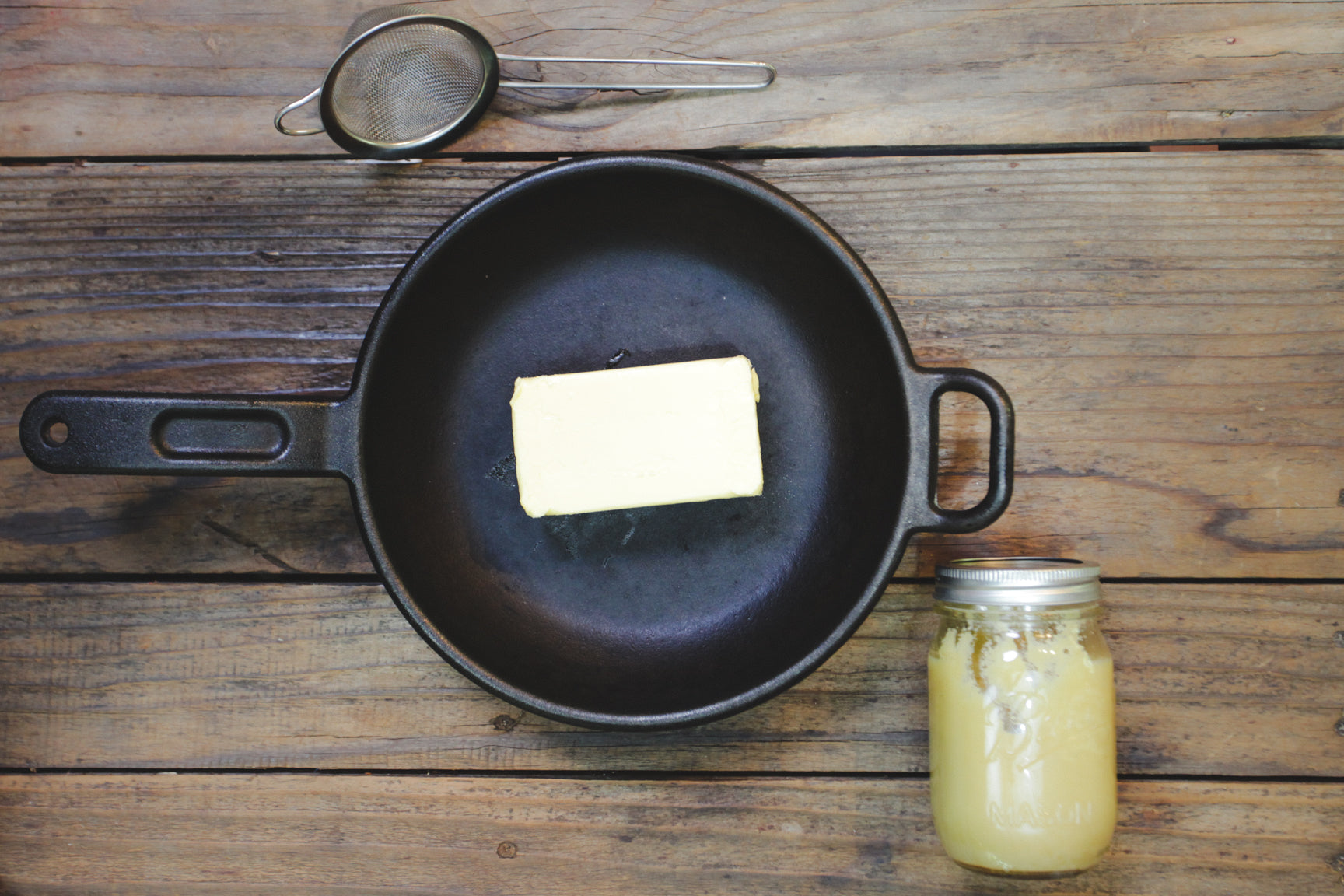On a dark brown wooden table, a black cast iron skillet sits prominently, photographed from above. The skillet features a handle on the left side with a hole for hanging and another smaller handle on the right. Inside the skillet is a large, yellowish-white chunk of butter, roughly the size of two sticks combined. Situated to the bottom right of the skillet is a glass mason jar with a silver metal lid, containing a creamy white substance, possibly lard or old grease. At the top left of the skillet lies a small, silver strainer with a long handle, suggesting it might be used to strain the butter into the jar. The setup is simple yet detailed, devoid of any text or additional activity, creating a focused and rustic scene.